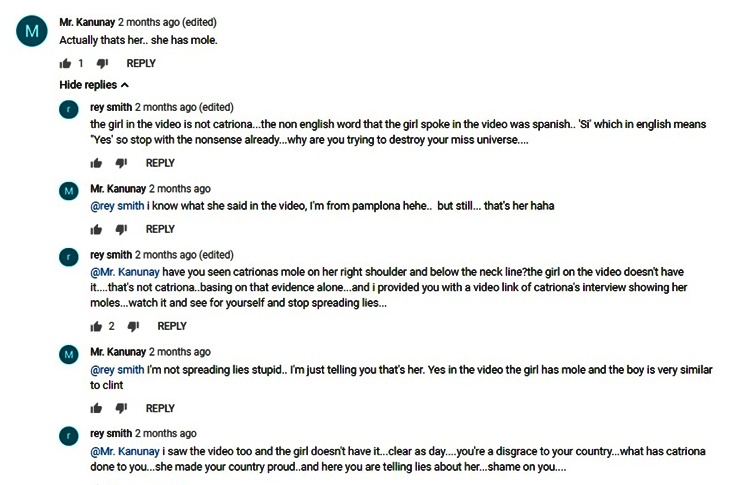**Caption:** 

Mr. Kananui and Ray Smith engage in a heated discussion about the identity of a girl in a video. Mr. Kananui asserts that the girl is Catriona, despite editing and claims to the contrary, pointing out a mole as evidence. Ray Smith counters, noting the girl in the video spoke Spanish and lacks Catriona's distinctive mole on her right shoulder and below the neckline. He provides a video link of Catriona's interview for comparison. The argument escalates with accusations of lying and disrespect towards Catriona, emphasizing her contributions to national pride.